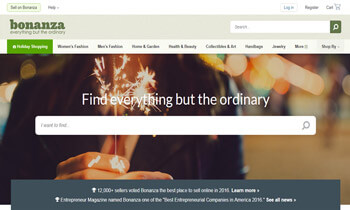The image is a small screenshot of the Bonanza website. In the upper left-hand corner, the Bonanza logo is prominently displayed in green font within a light gray header box that spans the width of the image. On the right side of this gray header, there is a search bar featuring a green button with a white magnifying glass icon, serving as the search function. Directly below this header is the main navigation menu, which consists of 10 distinct options. Centered in the main window, the large white text boldly states, "Find everything but the ordinary." Beneath this phrase is an expansive white search bar that dominates the middle portion of the screen.